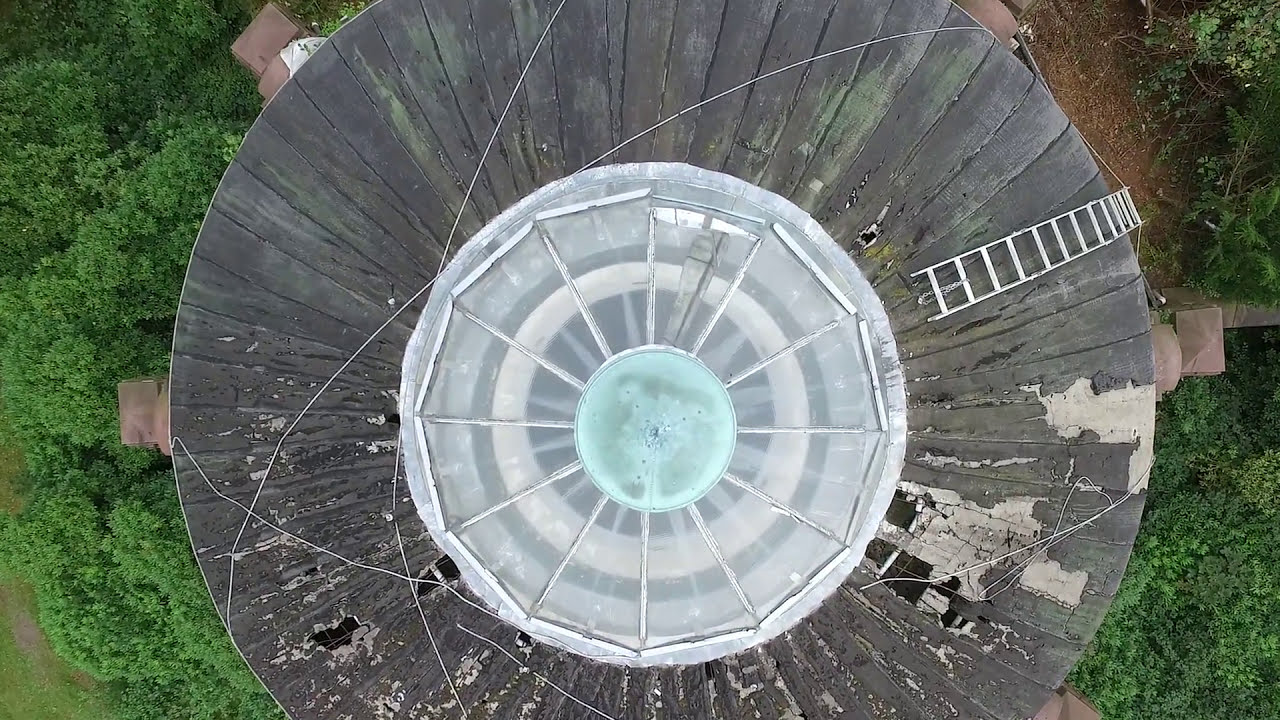This photograph captures a bird's eye view of a deteriorating, circular wooden roof, likely the top of a lighthouse. The roof is composed of dark, possibly black or dark brown wooden planks, many of which are peeling, breaking apart, and showing signs of significant wear. A white ladder lies on top of the roof, leading towards the center where there is a large, transparent, glass window with multiple concentric circles within it, possibly part of the lighthouse's light mechanism. Strewn across the roof are various wires and cables. Below, the landscape features a dense spread of bright green treetops, interspersed with patches of brown dirt and green bushes, reinforcing the natural surroundings of the structure.